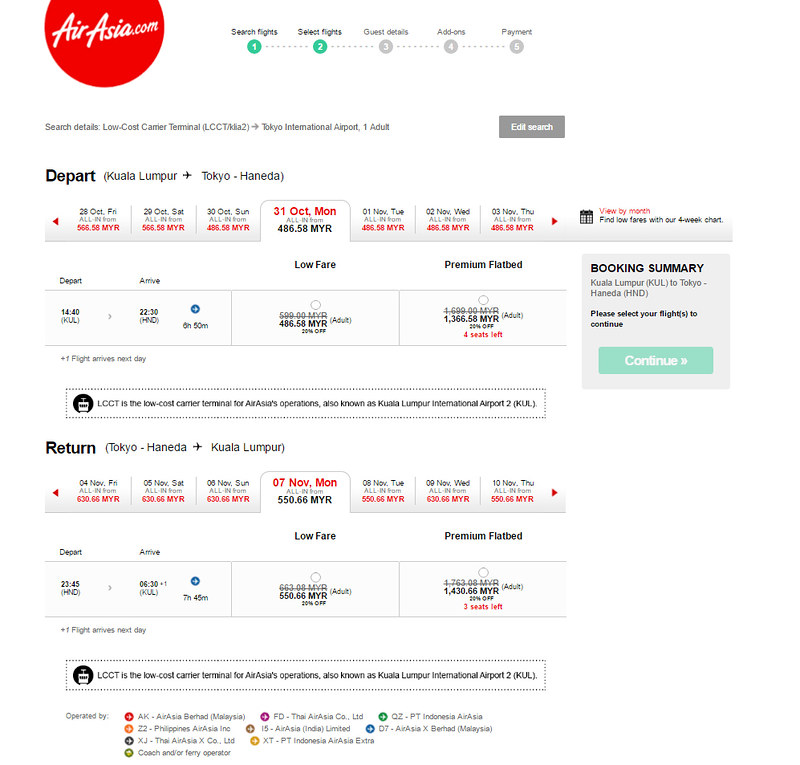A screenshot from the official AirAsia website is presented, featuring a structured layout for booking a flight. The title "AirAsia.com" is prominently displayed with both 'A's capitalized. The user interface showcases a five-step booking process: 1) Search Flights, 2) Select Flights, 3) Guest Details, 4) Add-Ons, and 5) Payment.

The search details section begins with the term "Low-Cost Carrier Technical" abbreviated as LCCT/MA2. The origin is Kuala Lumpur International Airport (abbreviated as LCCT) and the destination is Tokyo International Airport (Haneda - HND). The search is configured for one adult passenger with an option to edit the search. 

Below this, the departure information is listed: flying from Kuala Lumpur (depicted by an airplane icon) to Tokyo Haneda (HND). A comprehensive booking summary is positioned on the right side, highlighting key journey details and featuring a prominent green "Continue" button. The screen is designed to assist users in navigating through the booking process, with all pertinent information such as departure, return details, and the option to "Edit Search" located at the top right for user convenience.